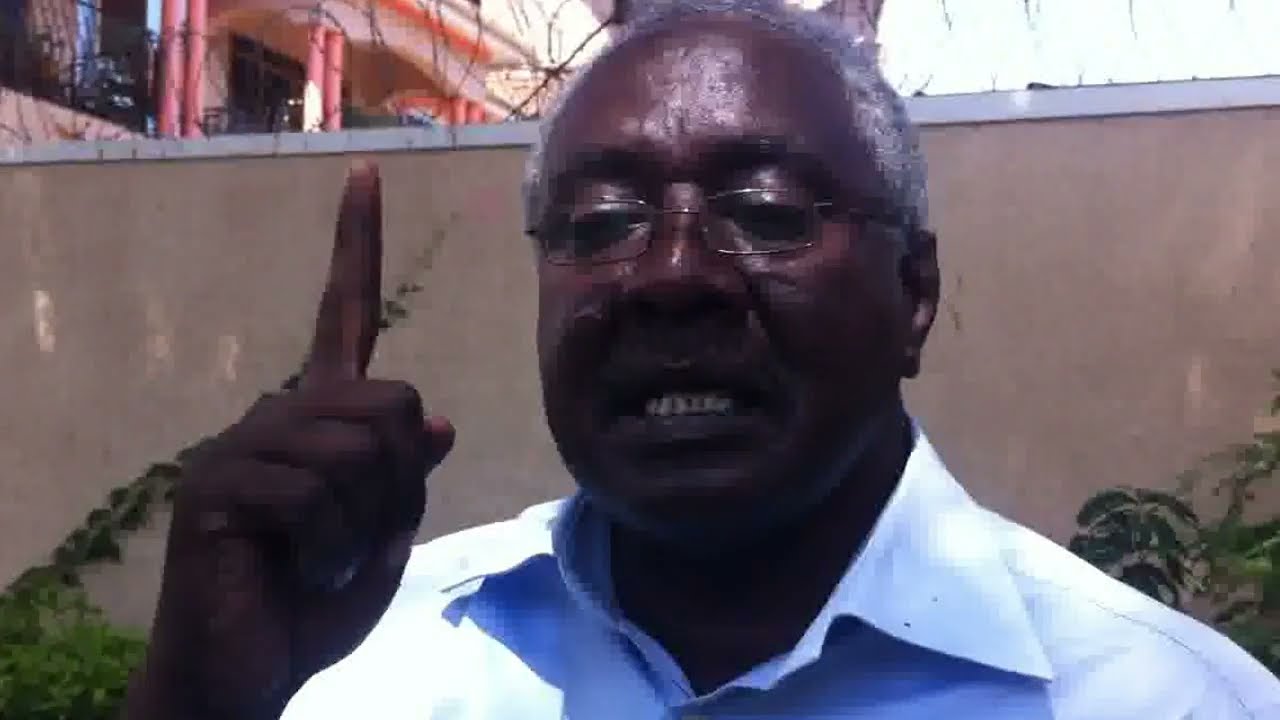The image features a close-up of an older African-American man with very dark brown skin and very short, white hair, balding on top. His face is partly shadowed due to poor lighting, with bright light highlighting his shiny forehead. He is at the center of the horizontally-oriented photo, wearing thin, silver-rimmed glasses. His mouth is open, with only the bottom row of his clenched teeth visible. The man is raising his right hand in front of his face, pointing his forefinger straight up, as though making a gesture. He dons a collared shirt, either white or light blue; the exact color is difficult to determine due to blurriness. 

In the background, there is a tall, beige wall with a white top ledge. Green plants grow halfway up this wall, with one particularly noticeable sprig of ivy extending diagonally upwards. To the upper left, a salmon-pink building with cylindrical pillars is partly visible. The sky in the upper right appears bright and white. The overall clarity of the photo is somewhat compromised, adding to the evocative quality of the scene.